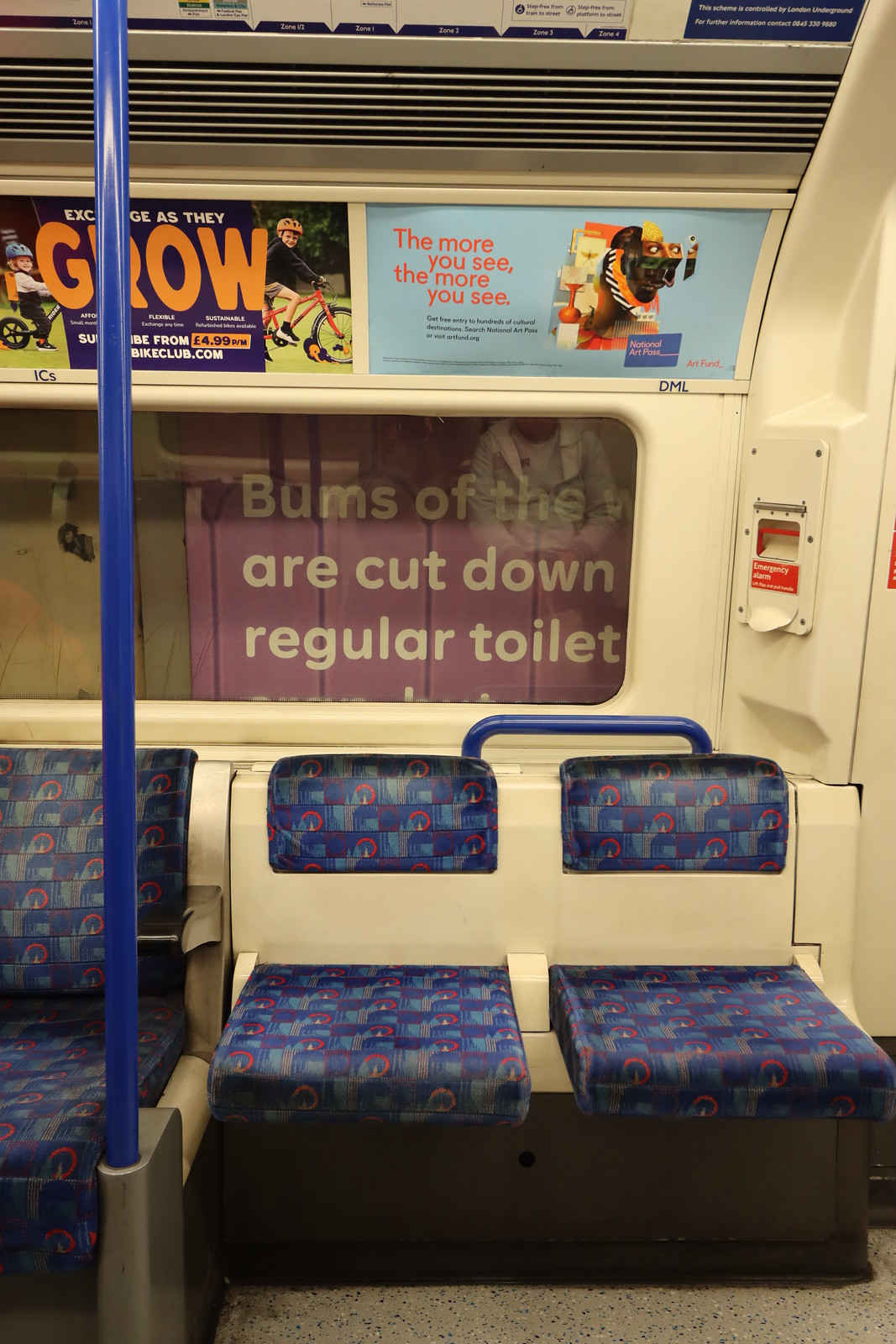The interior of a bus is prominently displayed, featuring seats upholstered in a distinctive blue and red box pattern. The first two seats visible in the foreground are single-person seats with a notable two-part design: a bottom cushion in the patterned fabric and a metal off-white segment that extends across both seats, followed by an upper cushion for back support. 

Adjacent to these, there is another seat which appears unclear in size but lacks the metal segment, showing only the patterned bottom and back cushions. In the background, a large window exposes an advertisement partially visible, reading, "bums of the are cut down regular toilet," hinting that the full ad is outside the bus.

Above the seats, two more advertisements are visible. One features a large text in orange, reading something about children growing, accompanied by an image of a young boy on a bike wearing a helmet, and another child, also wearing a helmet, on a bike or tricycle. Next to this, a cryptic advertisement states, "the more you see the more you see," with an obscure and odd image that appears to depict a half-dog, half-person figure. The overall scene is both colorful and somewhat peculiar, marked by incomplete advertisements and intriguing patterns.